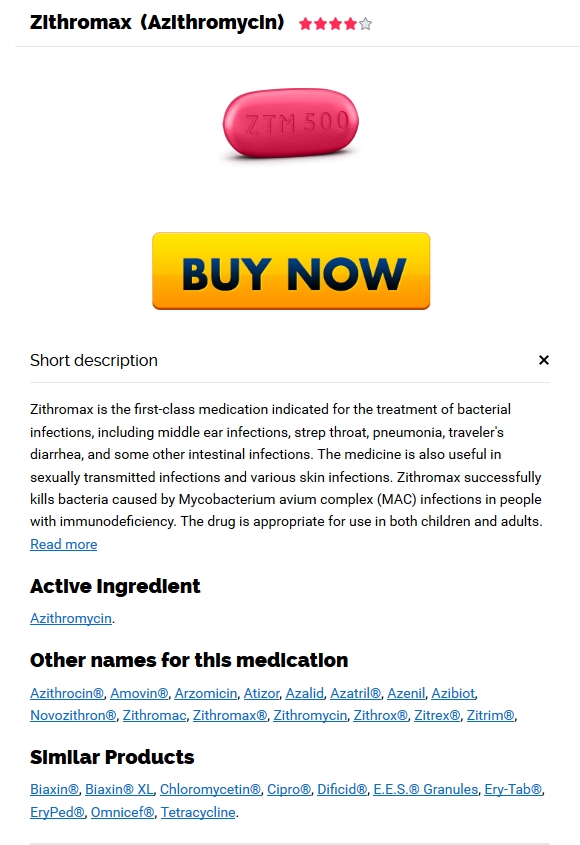### Detailed Caption:

**Zithromax (Azithromycin) - 500 mg**

This is an image of three Zithromax pills, each of which contains 500 mg of the active ingredient, azithromycin. The pills are red in color with the imprint "18" on them. Azithromycin, marketed as Zithromax, is a first-class medication primarily prescribed for the treatment of various bacterial infections. These conditions include middle ear infections, strep throat, pneumonia, and childhood diarrhea, among other intestinal infections. Additionally, Zithromax is effective in treating sexually transmitted infections and various skin infections. It is especially beneficial for people with immunodeficiency as it can combat infections caused by Mycobacterium avium complex. Suitable for both children and adults, this medication has a broad spectrum of antibacterial activity.

**Alternative Medications:**
- Asimovirin
- Azmovirin
- Azithrilazine
- Azobatin
- Novozithron
- Citron
- Psiloponics
- Biaxin
- Baxonexal
- Chloramaya
- Citrin
- Cipro
- Tuscanulose
- Tetra